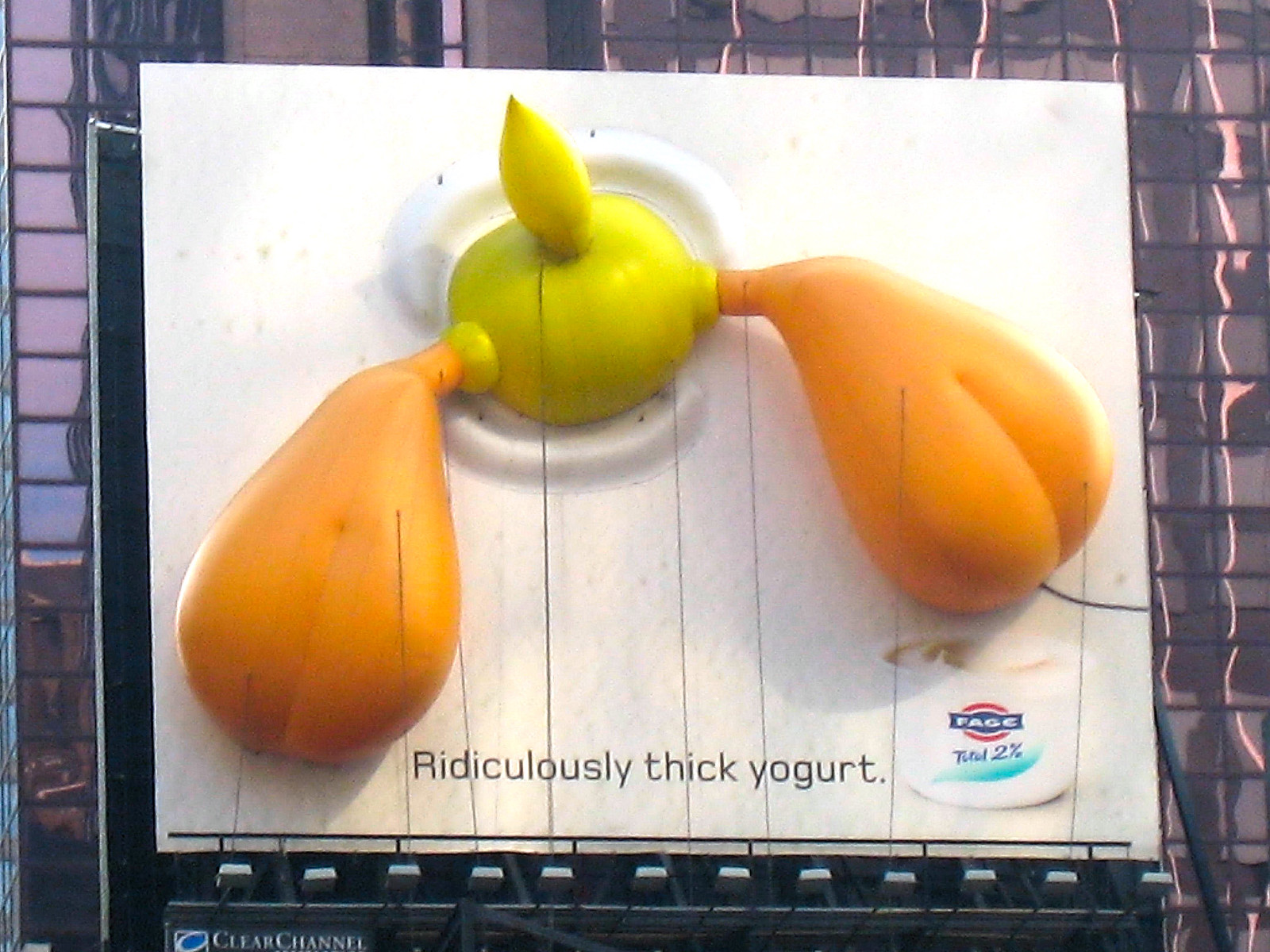This amusing image features a colossal billboard mounted on the side of an enormous building, accentuated by twelve light fixtures at its base. Each light, approximately two feet wide, is separated by three-foot gaps, creating a symmetrical and visually engaging bottom frame. On the left bottom corner of the billboard, the "Clear Channel" symbol can be observed.

The building itself, housing the billboard, boasts around 15 rows and columns of windows, emphasizing its massive scale. The billboard’s design is striking with a white background that resembles yogurt. The text on the billboard reads, "Ridiculously Thick Yogurt," pointing to the product's rich consistency, with the brand name "FAGE" and "Total 2%" displayed prominently. 

Adding a humorous touch, the focal point of the billboard is a 3D duck seemingly submerged in the yogurt. The duck's yellow rear end and tail, along with its sizable orange feet, protrude from the billboard, creating a lifelike effect. The feet are affixed with strings tethered to the bottom and ankles, enhancing the three-dimensional illusion and making it appear as though the duck is actually stuck in the yogurt. In the bottom right corner of the billboard, a small tub of the yogurt further reinforces the advertisement, blending clever marketing with engaging visual art.